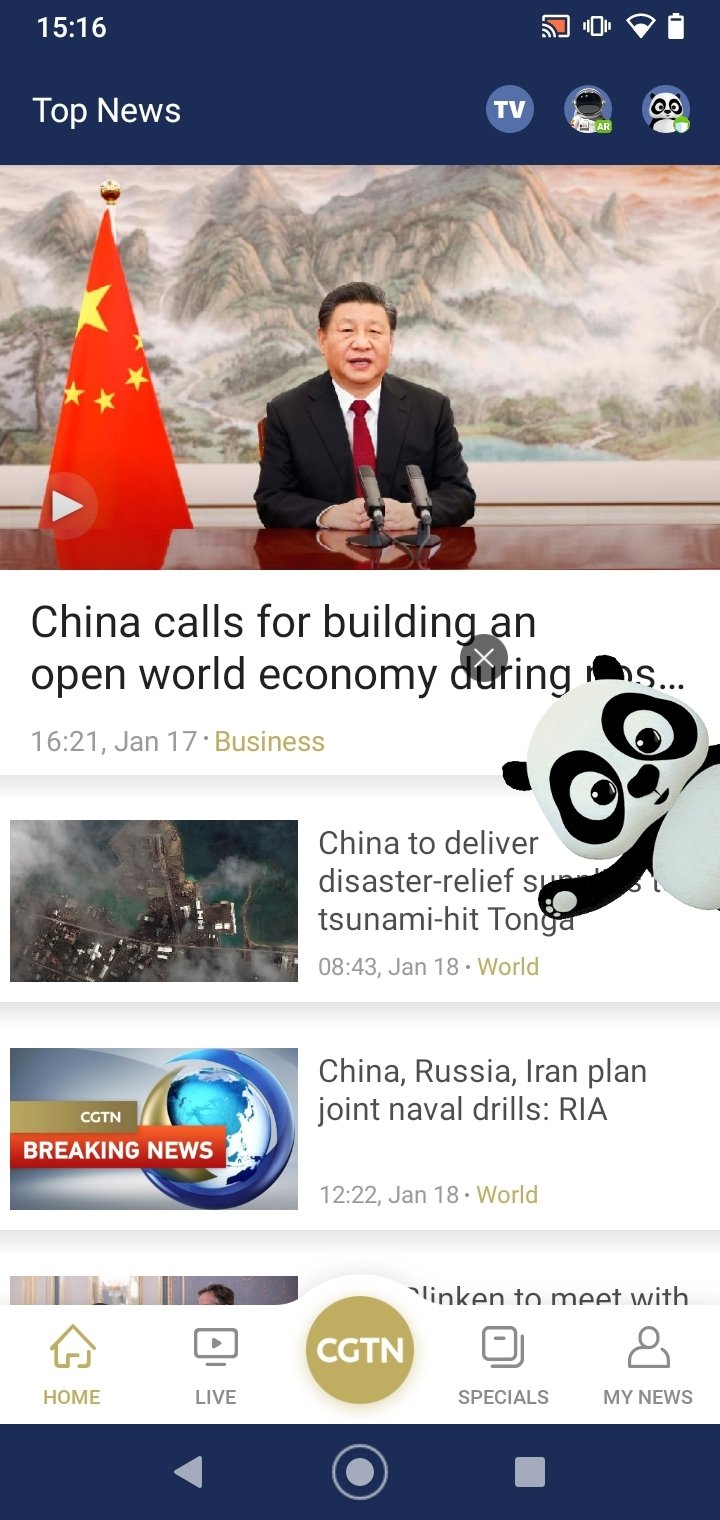Here is a cleaned-up and detailed caption for the image:

---

This screenshot features a header with a dark blue background and white text at the top. The time displayed is 15:16 on the upper right corner, along with a partially lit Wi-Fi icon and a full battery indicator. Directly below the header, the section labeled "Top News" includes three icons arranged horizontally on the right: the first icon is labeled "TV," the second shows the image of an astronaut's head with the letters "AR" in a green box, and the third is a cartoon character of a panda bear. 

Below the "Top News" section is a color photograph capturing an Asian man with black hair seated behind a shiny dark desk, with two microphones placed in front of him and his hands crossed. To his right, there is a Chinese flag, and behind him, a mural depicting mountains shrouded in fog. The text beneath this image reads: "China calls for building an open world economy during."

Additionally, emerging from the right side of the screen is another cartoon panda bear. Below this, the headline states: "China to deliver disaster relief surplus to tsunami-hit Tonga." The specific details of the article, including the time "08:43" and the date "January 18th," are also visible.